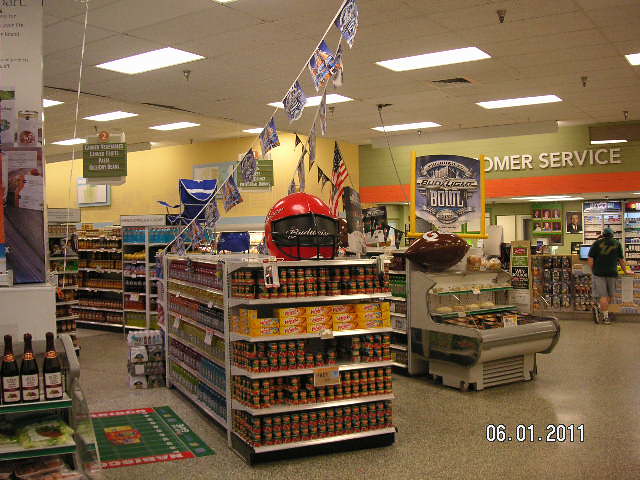Captured on June 1st, 2011, this photograph depicts a bustling store environment. At the forefront, a customer patiently waits to be assisted at the customer service counter. Surrounding them, various products are neatly arranged on shelves, including noticeable items like Velveeta cheese and cans of an indistinguishable tomato product. Featured prominently atop an end cap displaying these items, a striking red and black oversized helmet adds a unique touch to the shelf. To the right, a refrigerated case stands, crowned by an enormous inflatable football, suggesting a football season theme. The store's interior is vibrant with yellow and green walls and a variety of other shelves filled with merchandise. Above, the ceiling appears to be lowered, contributing to the cozy atmosphere of the store.